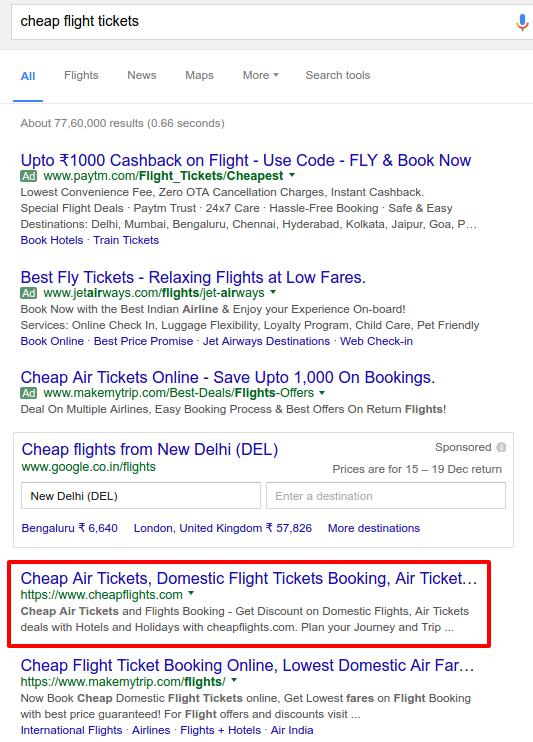**Detailed Caption:**

The image is a screenshot of a Google search results page with the query "cheap flight tickets" entered in the search bar. At the top of the page, there are several navigational tabs labeled: "All," "Flights," "News," "Maps," "More," and "Search tools." Just below the tabs is a grey separating line, indicating that the search yielded about 77,060,000 results in 0.66 seconds.

The first entry at the top is a highlighted advertisement offering up to $1,000 cashback on flights with a promotional code "FLY" and an encouragement to book immediately. The next listing promotes "Best Fly Tickets" from Jet Airways, featuring relaxing flights at low prices. This is followed by another entry from MakeMyTrip.com, announcing cheap air tickets online with savings of up to $1,000 on bookings. The subsequent result is from Google Flights, displaying options for cheap flights from New Delhi. In a boxed area below this, there's an "Enter Destination" text field, with example destinations like Bengaluru (₹6,640) and London, United Kingdom (₹57,826), along with a prompt to view more destinations.

Further down the page, an entry within a red-outlined box advertises cheap air tickets for domestic flights from CheapFlights.com. The final result mentions low-cost flight booking with the lowest domestic airfares available on MakeMyTrip.com.

Overall, the search results consist primarily of advertisements and aggregate flight booking sites, providing various options for finding affordable airfare.